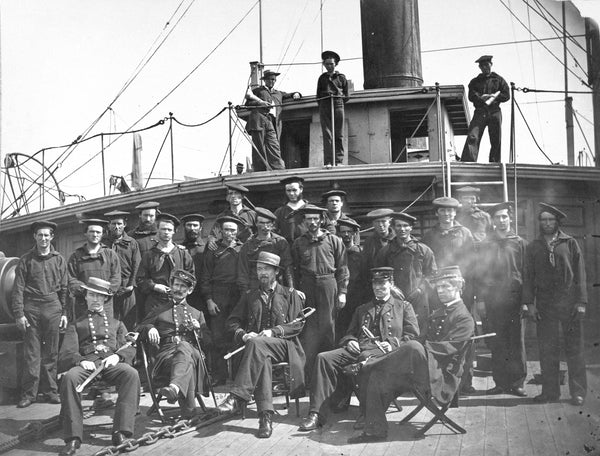This is an old black and white photograph depicting the crew of a naval ship, possibly dating back to the early 20th century, pre-World War I or II. The photograph captures at least a dozen men, with the majority standing on a lower deck and a few on an upper deck, all posing for what appears to be a formal crew photo. The men are attired in dark, simple military uniforms with sailor caps, suggesting they are sailors.

At the bottom of the image, five high-ranking men are seated in chairs. These seated men wear more elaborate uniforms adorned with numerous golden buttons, indicating their rank. Each of these men is equipped with a sword, albeit in different positions. The leftmost seated man holds a unique straw-like hat and has his sword laid across his lap. The man next to him has his sword with the hilt on the ground and his hand resting on it. The central seated man also has his sword across his lap, similar to the first. The man to his right has his sword resting against his thigh without touching it. Finally, the rightmost seated man's sword has the blade pointing behind him with the hilt on his lap.

In the background, the sky above the ship appears uniform in color, suggesting either a clear day or overcast conditions, though the exact weather detail is indistinct due to the photograph's monochromatic nature. Overall, the photograph presents a striking historical snapshot of naval life, capturing both the hierarchy and the camaraderie of the ship's crew.